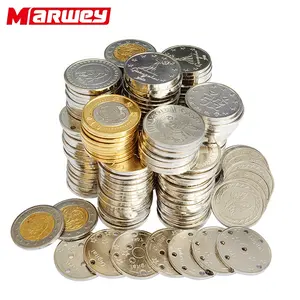The image features an assortment of various coins on a plain white background, emphasizing their details and arrangement. Most of the coins are meticulously stacked, while a few are scattered in a line at the front. These coins are quite diverse, showcasing different designs and features. Some have gold edges with silver centers, while others have the reverse—silver edges with gold or coppery centers. A few coins have darker spots or little dots on their surfaces, adding texture to their shiny, yet somewhat rough exteriors. Notably, some coins display Japanese characters. In the upper left corner of the image, there is a striking red logo that spells out "M-A-R-W-E-Y," with the 'M' in red and the 'RWEY' in white, set against the red background. The entire composition highlights the unique characteristics and international origins of the coins.